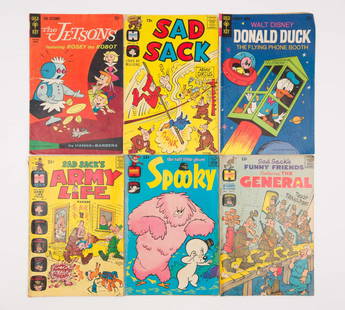The image is a color photograph of six vintage comic book covers arranged in two rows and three columns, each comic vertically rectangular with a light gray border around the entire collection. In the top left corner is *The Jetsons*, featuring a red cover with white lettering; prominent characters include Rosie the Robot, George, Jane, and Elroy. The middle comic in the top row is titled *Sad Sack*, set against a yellow background with red and blue text, depicting people attempting a pole vault. The top right comic is *Donald Duck*, which has a blue background showing Donald Duck trapped inside a flying telephone booth with an alien nearby. Moving to the bottom row, the leftmost comic is *Army Life*, which displays several men and a dog against a yellow background. The center comic on the bottom row is *Spooky*, showcasing a small white ghost wearing a hat next to a pink monster, all set against a blue background. Finally, the bottom right comic is titled *Funny Friends of the General*, illustrating people standing on a beam.

This descriptive caption synthesizes common elements from all three versions, highlighting shared details and providing a clear, comprehensive visual guide of the image.